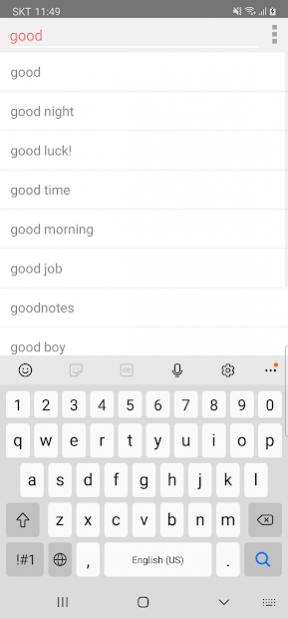The image displays a user's smartphone screen, depicting search results. At the very top, a dark gray status bar shows the time as 11:49, a notification bell icon with a line through it (indicating notifications are off), a fully charged battery icon, and no bars for signal strength. The label "SKT" is adjacent to the time.

Below the status bar, there is a light gray search bar with the word "good" highlighted in red. Following this are a series of search suggestions presented in a vertical list: "good," "good night," "good luck!" "good time," "good morning," "good job," "GoodNotes," and "good boy." Each suggestion is neatly organized in a separate row.

At the bottom of the screen is a keyboard, starting with a row of numbers at the top. Above the numbers, there are icons for an emoji, a microphone, settings, and three dots for additional options. The main keyboard, which is typical for text input, follows the number row. In the lower right-hand corner of the keyboard, a bright blue magnifying glass icon indicates the search function.